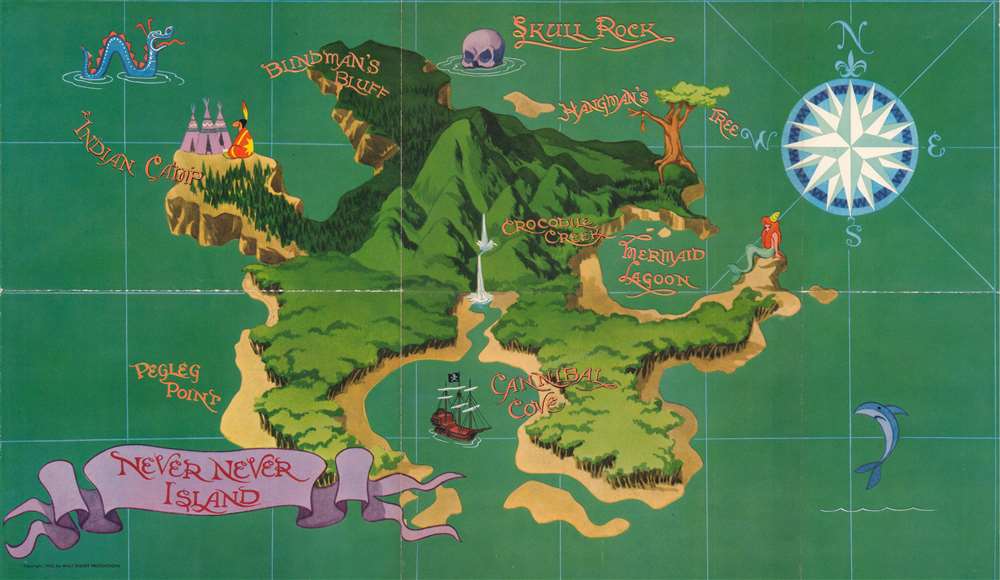The image depicts a fantastical and intricately illustrated map of "Never Never Island," characterized by its vibrant and modern style with a touch of vintage charm. Prominently labeled landmarks like "Blind Man's Bluff," "Indian Camp," "Peg Leg Point," and "Mermaid Lagoon" suggest a rich narrative backdrop. A detailed compass rose adorns the upper right corner, indicating the cardinal directions. The island itself is surrounded by a teal-hued sea and is dotted with diverse terrains, including green forests and prominent mountains. Notable features include a ship navigating towards a cove, a solemn figure beside a teepee, a swimming dragon, and a striking skull rock in the middle of the water. The island's purple highlights capture attention amidst predominantly green tones, and whimsical elements such as a red bird perched on a peak and a blue dolphin frolicking in the sea add to the enchanting atmosphere. Overall, the map exudes a sense of adventure and fantasy, likely intended for a children's storybook.